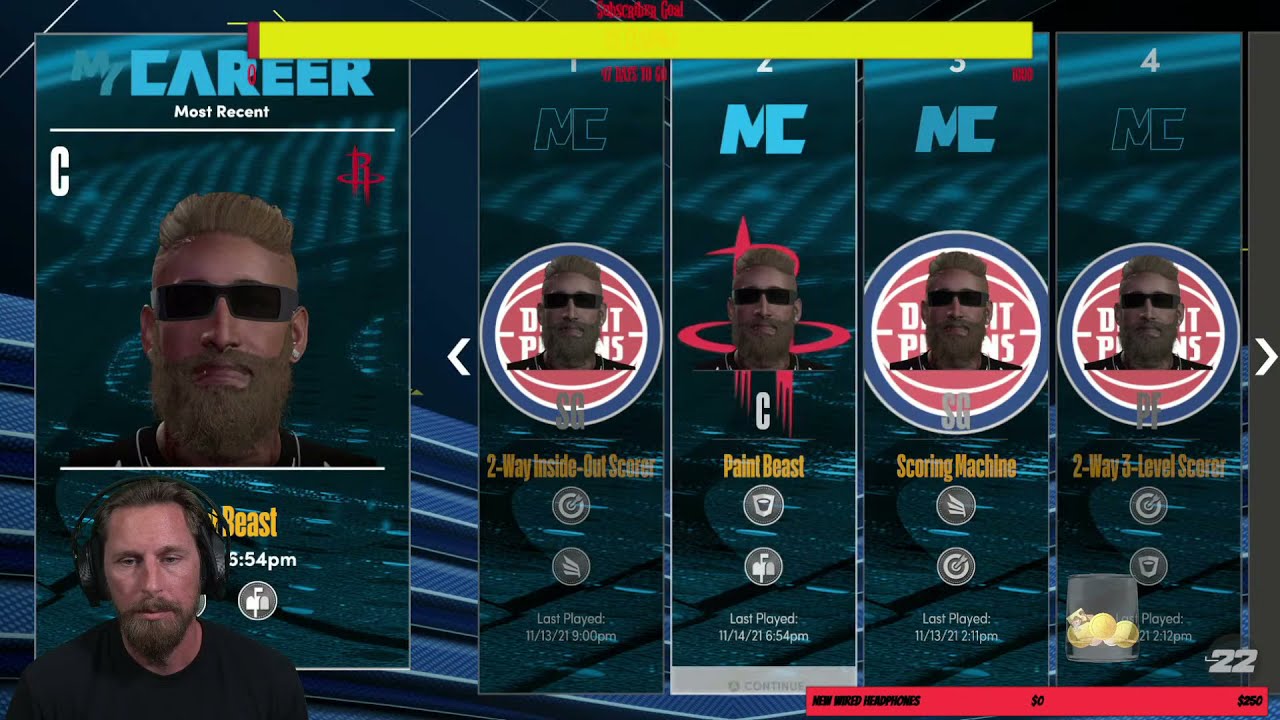The screenshot captures a Twitch stream of a man playing the video game 2K22. In the bottom left-hand corner, the streamer, a man in his late 30s to mid-40s with light brown hair, a thick beard, and a mustache, is visible. He is wearing a black t-shirt and over-the-ear headphones, facing slightly downwards. Behind him, the game's interface is displayed prominently. On the upper left corner, the text "My Career" and "Most Recent" is visible above a square photo of a man with blonde spiked hair, a thick beard, and black sunglasses, which appears to be the player's avatar.

The center of the screenshot features four columns, each labeled 1, 2, 3, and 4, with the letters "MC" beneath the numbers. In each column, the same avatar appears inside blue and red circles, with various titles underneath, such as "Two-Way Inside Out Scorer," "Paint Beast," "Scoring Machine," and "Two-Way Three-Level Scorer." The avatars are displayed against alternating backgrounds featuring the logos of the Houston Rockets and the Detroit Pistons. The overall color scheme includes blue, red, and black elements, and in the bottom right-hand corner, a red bar with some words is partially visible, along with the number "22," indicating the game is 2K22.